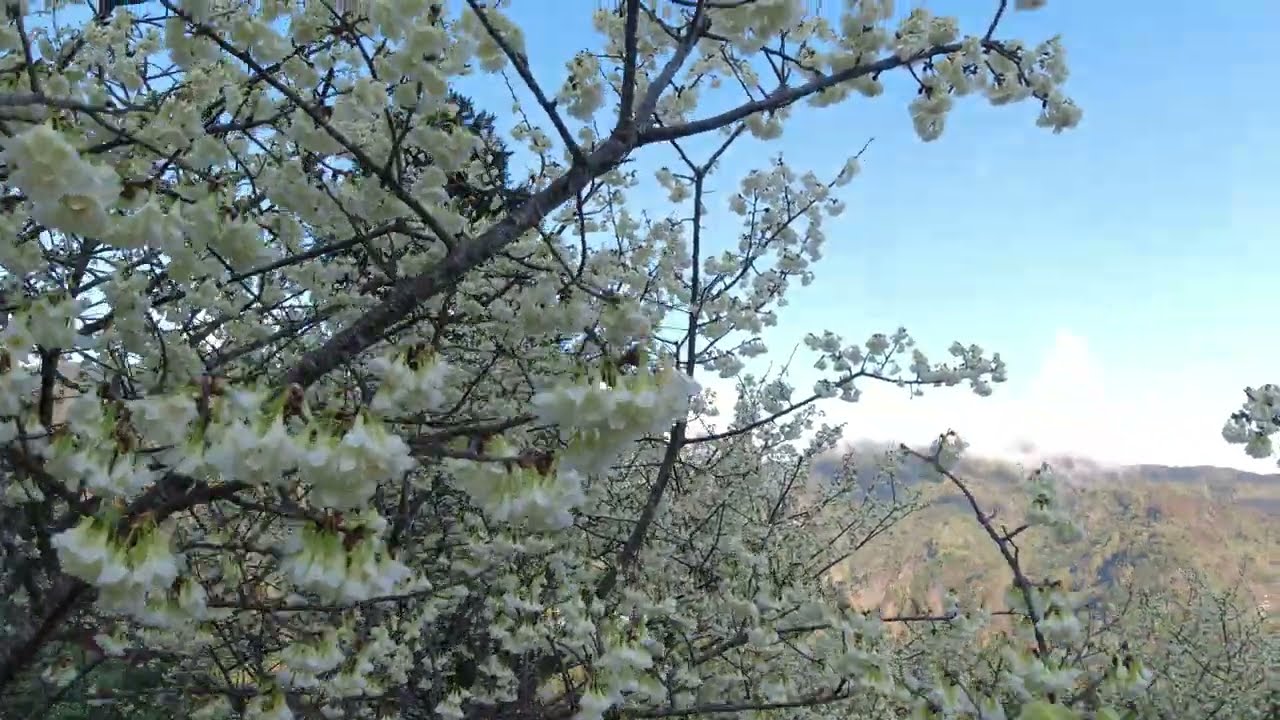The image depicts a vibrant outdoor scene dominated by a partly cloudy blue sky that transitions to a lighter white hue near a distant mountain range. The foreground is filled with numerous branches adorned with an abundance of small, white flowers, suggesting it could be early spring or late fall. These branches, with thin, bright green stems and a hint of dark brown bark, extend from the left side and occupy about two-thirds of the frame, leaving the upper right corner more open to highlight the expansive sky. Scattered throughout the bottom of the image, a few more branches can be seen, blending into the more distant vegetation that appears to shift from green to brown. The scene's details, including what looks like possibly prickly branches and densely packed flower clusters, give the impression of a blooming tree or bush seen from a slightly elevated perspective, emphasizing the contrast between the lush foreground and the serene, mountainous background.